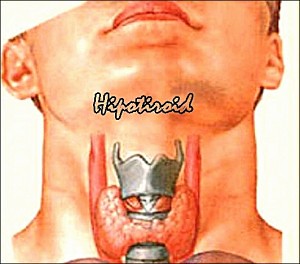This detailed anatomical drawing depicts a section of a man's face and throat presented on a tan background. The man's head is tilted upward, showcasing his chin, lips, and ears, with the primary focus on the throat area. The drawing highlights internal structures within the throat, featuring two red, stem-like lines running upwards from a round, red object situated at the throat's center. This object appears to have a metallic or silver cap atop it. Below this cap are metallic-looking elements that resemble parts of the spinal column. The text “HYPOTYROID” is prominently displayed in white cursive letters outlined in black above the anatomical details.